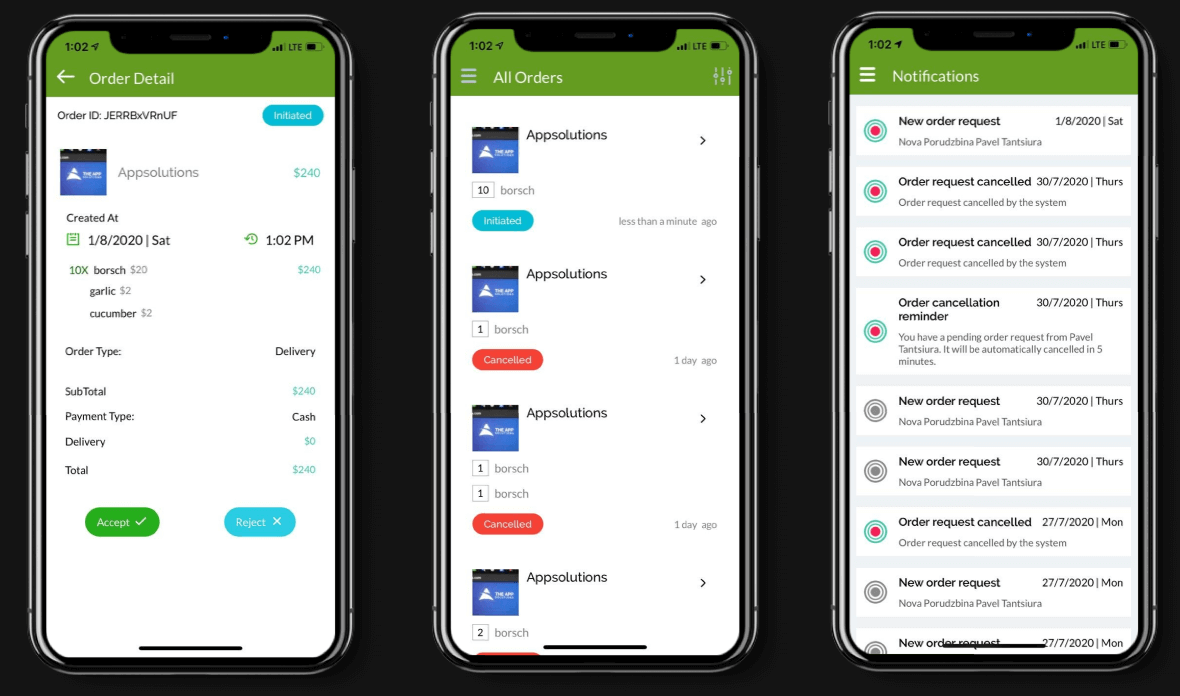The image features a sleek black background with three smartphones placed side-by-side. Each smartphone has a distinct display and a dark green border at the top, giving them a unified appearance.

The screen of the smartphone on the left shows an 'Order Detail' page with an arrow pointing to the left. Below that, it displays an order number "App Solution 9240," created on January 8, 2020, at 1:02 p.m. The details include a menu listing various vegetables, as well as information about the payment method, delivery details, and the total price of the order.

The middle smartphone exhibits a layout featuring four blue icons, each accompanied by the label "App Solution." These icons are likely representing different functions or sections of the app, providing a user-friendly interface.

The smartphone on the right showcases a series of notifications about order requests. The top notification states "New Order Request," followed by notifications for "Order Request Cancelled," "Order Cancellation Reminder," and another "Order Request Cancelled."

Overall, the image portrays a comprehensive view of an app interface focusing on order management and notifications, framed by a sophisticated black background.